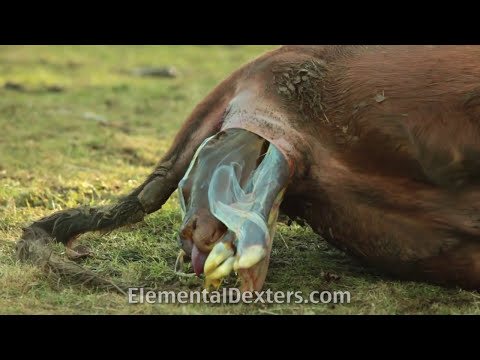In this detailed image, a large brown cow is lying down in a field of short grass, giving birth to a calf. The focus is on the rear of the cow, which is situated towards the right side of the image; the left side is predominantly grass. The cow has mud crusted on its tail and rear flank. Emerging from the cow's rear, the head and hooves of the calf are visible, with the tongue of the calf sticking out and enveloped in an amniotic sac. Colors present in the image include shades of black, green, lime green, yellow, brown, and tan. The scene is set against a completely black background, emphasizing the birth process in this outdoor, possibly educational, setting. Below the image is the text "ElementalDexters.com," likely indicating the source or context of the photograph.